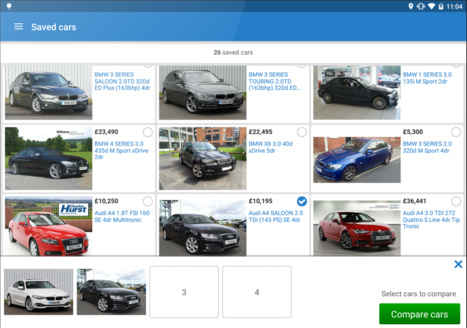The image is a screenshot of a website displaying vehicles for sale. At the top of the webpage, there is a dark blue-colored navigation bar which includes icons on the upper right: a GPS icon, a vibration icon, a battery life indicator, and a Wi-Fi signal icon. Additionally, the current time displayed is 11:04. 

Beneath the navigation bar, a header with a blue background shows "Saved Cars" written in white font, indicating that the user has saved 26 cars to their list. Below this header, the webpage lists detailed information and images of various saved vehicles. 

The list includes:
1. BMW 3 Series Saloon 2.0 TD 320d ED Plus
2. BMW 3 Series Touring 2.0 TD
3. BMW 1 Series 3.0 I 135i M Sport
4. BMW 4 Series 435d M Sport xDrive, priced at £23,490
5. BMW X6 45d xDrive 5dr, priced at £22,495
6. BMW 3 Series 2.0 320d M Sport, priced at £5,300
7. Audi A4 1.8 FSI 160 SE, priced at £10,250
8. Audi A4 Saloon 2.0 TDI, priced at £10,195
9. Audi A4 3.0 TDI 272 Quattro S-Line, priced at £36,441

At the bottom of the list, there is a green button labeled "Compare Cars," allowing users to compare selected vehicles side by side.